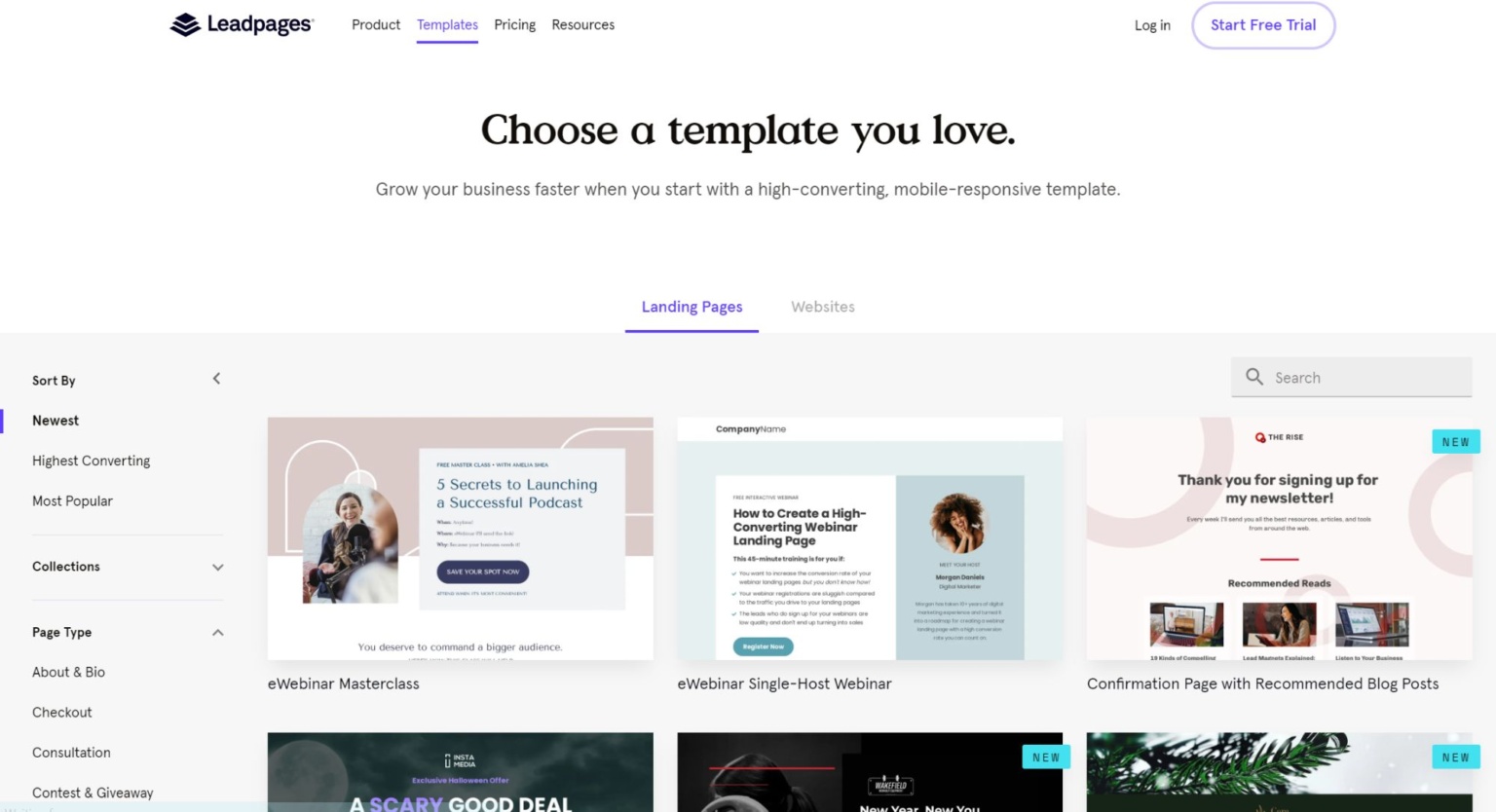**Caption:**

Screenshot of a LeadPages website showcasing template options. The top banner features the LeadPages logo. The page title, "Choose a Template You Love," is prominently displayed, followed by a description emphasizing the benefits of high-converting, mobile-responsive templates for business growth. 

Below the description is the beginning of a template grid set against a light gray background. The grid displays three landing page options per row, with only the first row fully visible. The visible templates include: "5 Secrets to Launching a Successful Podcast," "How to Create a High Converting Webinar Loading Page," and "Thank You for Signing Up for My Newsletter." The second row's leftmost template is titled "A Scary Good Deal," with the rest cropped out of view.

On the left side, a menu bar provides filtering options such as Newest, High Converting, Most Popular, Collections, Page Type, About and Bio, Checkout, and Consultation templates, facilitating easy navigation for users looking to create their own websites with LeadPages.